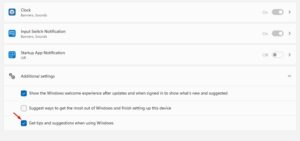In this image, we can see a clock icon prominently displayed, accompanied by several additional setting options. There is text present in the image, but it is heavily blurred and rendered illegible due to the poor quality. The text appears in varying colors, primarily blue and red. Certain items within the settings are automatically checked by default and cannot be deselected. At the bottom of the image, there are three checkboxes, with the first and third checkboxes marked as checked, while the center checkbox remains unchecked.